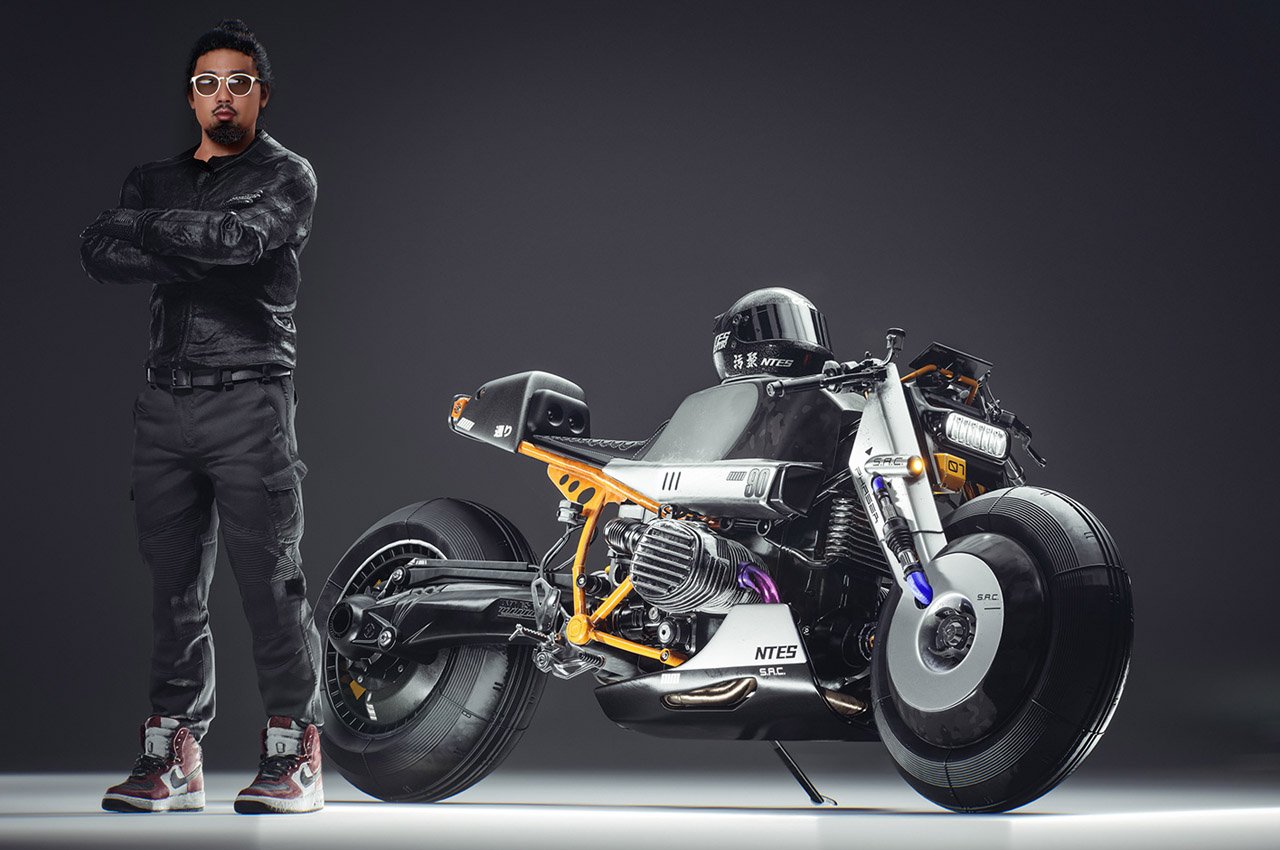The image features an Asian man, positioned on the far left, posing next to a futuristic-looking sports motorcycle. He has black hair tied into a short man bun, and he wears white-framed sunglasses and a black goatee. His outfit consists of a black leather biker jacket with a belt around his waist, black cargo pants, and a pair of Nike Air Jordan shoes in red, black, and white. The motorcycle, prominently displayed in the center, has a sleek, modern design with an orange, silver, and black body and large, black wheels. Resting on the gas tank is a black helmet, and the letters "NTSSAC" are visible on the side. The entire scene is set against a plain gray background.